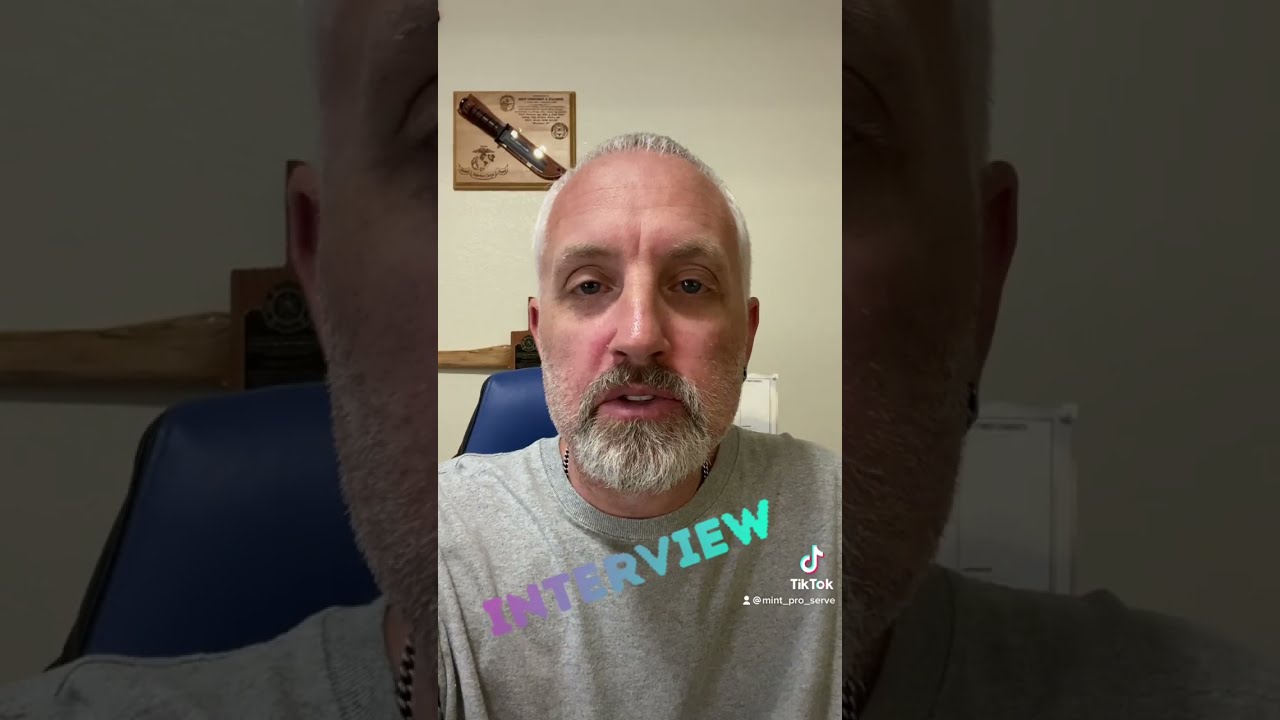The image appears to be a color screenshot of a cell phone screen capturing a TikTok video. It features an older Caucasian man with short, white hair and a matching goatee, along with a bit of white stubble. He has blue eyes and fair skin, and he is sitting directly in front of the camera on a blue chair. The man's outfit includes a light heather gray t-shirt and a silver chain tucked into the shirt. Text in ombre shades from purple to light blue, reading "interview," is angled across his chest, while the TikTok logo and the username "@Mint_pro_serve" are displayed on the right side of the image.

The background of the image consists of a beige wall, although it was previously noted as "white" in other descriptions. Hanging on the wall, above the man's head, is a K-Bar knife mounted on a brown wooden display case. This display features the Marine Corps emblem with an eagle, globe, and anchor, reinforcing its military nature. Below the display case, there appear to be some cabinets. The overall composition suggests the man is in a home setting, possibly recording a TikTok video about his experiences or interests.